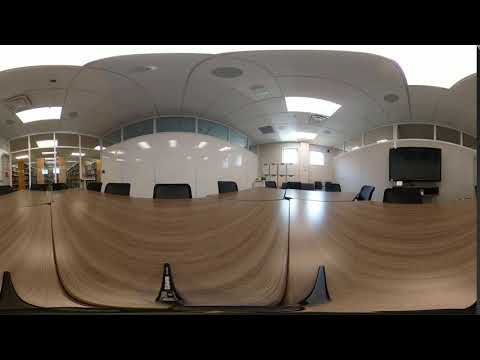The image depicts a corporate meeting room with a light beige wooden table extending across the center and surrounded by sleek black chairs. The room, captured with a 360-degree camera, appears slightly distorted due to the stitching of multiple images, giving it a curved, panoramic effect. The walls are shiny and white, contributing to a clean, modern ambiance. Notably, on the left-hand side, there are glass doors that reveal an adjacent room filled with bookshelves, reminiscent of a library. Also on the left, tall floor-to-ceiling glass windows bring in natural light. On the right side of the room, a flat-screen television is mounted on the wall with an accompanying device beneath it. The ceiling is white and features fluorescent lights, completing the well-lit and polished look of this corporate space.